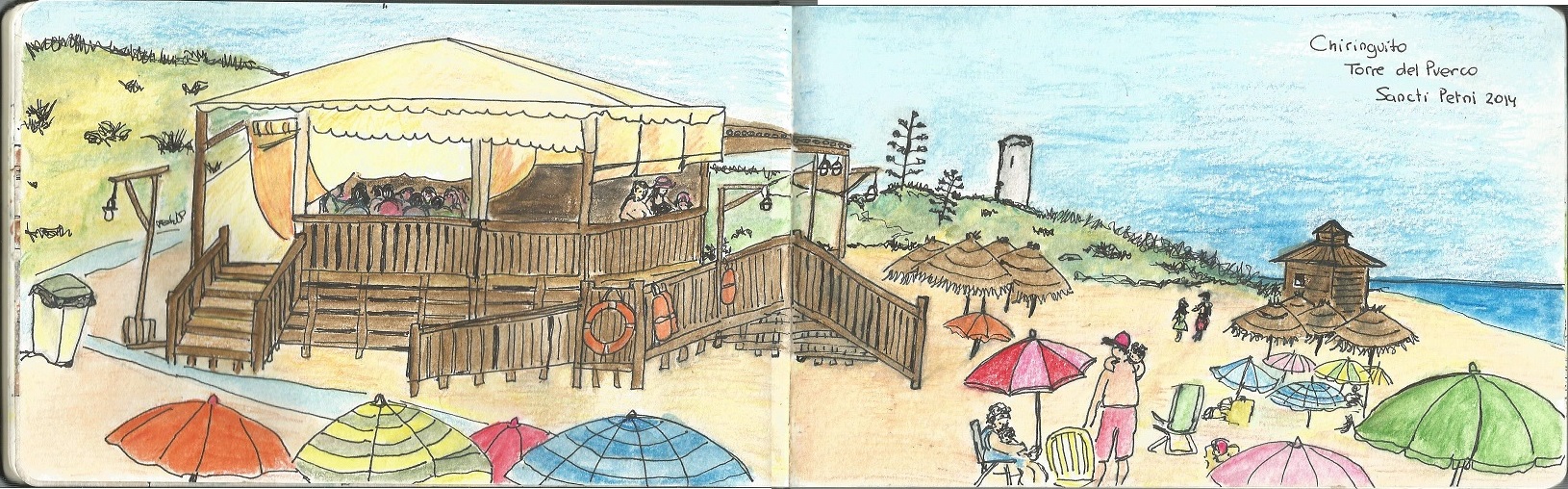Illustrated in vibrant, vivid colors, this detailed comic-strip style drawing captures a lively beach scene from a sketchbook spread. The beach is adorned with an array of colorful umbrellas in shades of pink, green, blue, yellow, orange, and varying hues of pink and red. Among the umbrellas are small huts that feature grass or wicker rooftops. Set against a backdrop of blue skies and green grass, a prominent wooden beach house with a yellow canvas roof and lifebuoys scattered around stands out. This beach house, accessible via a wooden ramp, has people inside, observing the scene around them. A man wearing red shorts and a red hat stands near the ramp, and there is also a person seated nearby, possibly holding a baby. A green trash can can be spotted at the edge of the drawing. The text "Chiringuito Torre del Puerco, Sancti 2014" is inscribed on the right side of the sketchbook, adding a title to this vibrant beach illustration.